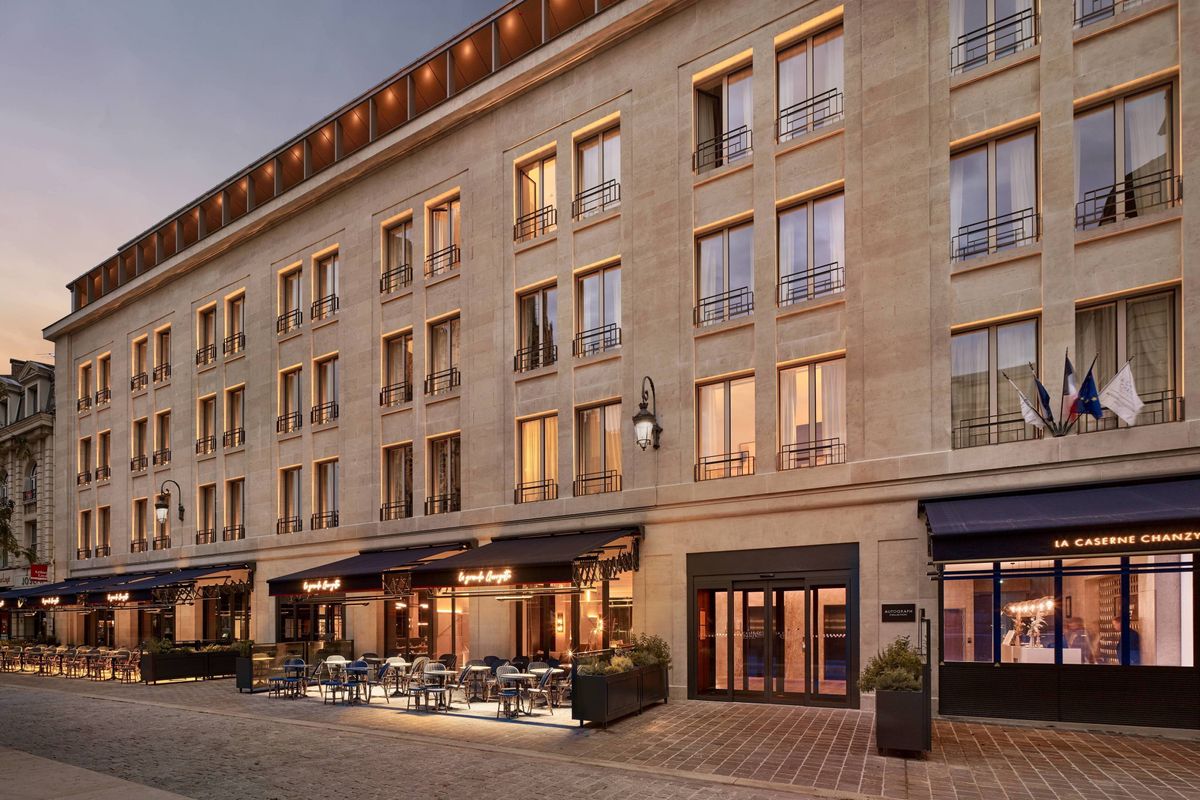The photograph depicts a sprawling four-story, grayish-beige building at dusk, illuminated by the soft evening light. This building is set in a European city and spans the entire width of the image, displaying a combination of residential and commercial use. The ground floor is composed of various storefronts, cafes, and restaurants, one notably named "La Casern Chanzy." Each storefront features black awnings with golden lettering, adding a touch of elegance. Above these shops, the building transitions into residential apartments, as evidenced by the repetitive patterns of double windows on the upper three floors. Each window is adorned with a black Juliet balcony or guard rail, and many windows have beige curtains. Black metal barring and striking gold-painted trims accentuate the windows, providing an aesthetically pleasing contrast. The upper portions of the building are outlined with glowing lights, adding to the twilight ambiance. The scene is completed by a cobblestone or tiled sidewalk lining the street, with several outdoor seating areas arranged for dining, indicating the vibrant yet cozy atmosphere of a busy urban center.